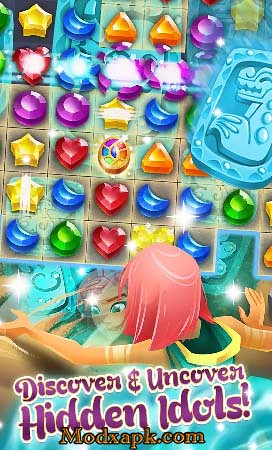The image shows a children's game named "Hidden Idols," displayed in vibrant purple letters at the top. The goal of the game, "Discover and uncover hidden idols," is prominently featured, though the manufacturer's name is not legible. Two children are depicted in the lower portion of the image: one with long, flowing hair that appears red or pink, facing away from the viewer, and another child looking towards her with large, expressive eyes reminiscent of Disney characters. Above the children, there is a game board adorned with a variety of multicolored, differently shaped symbols, which seem to be interactive elements that players must remove or press to uncover the hidden idols. A notable turquoise patch is situated on the right-hand side of the image, adding a pop of color to the overall scene.